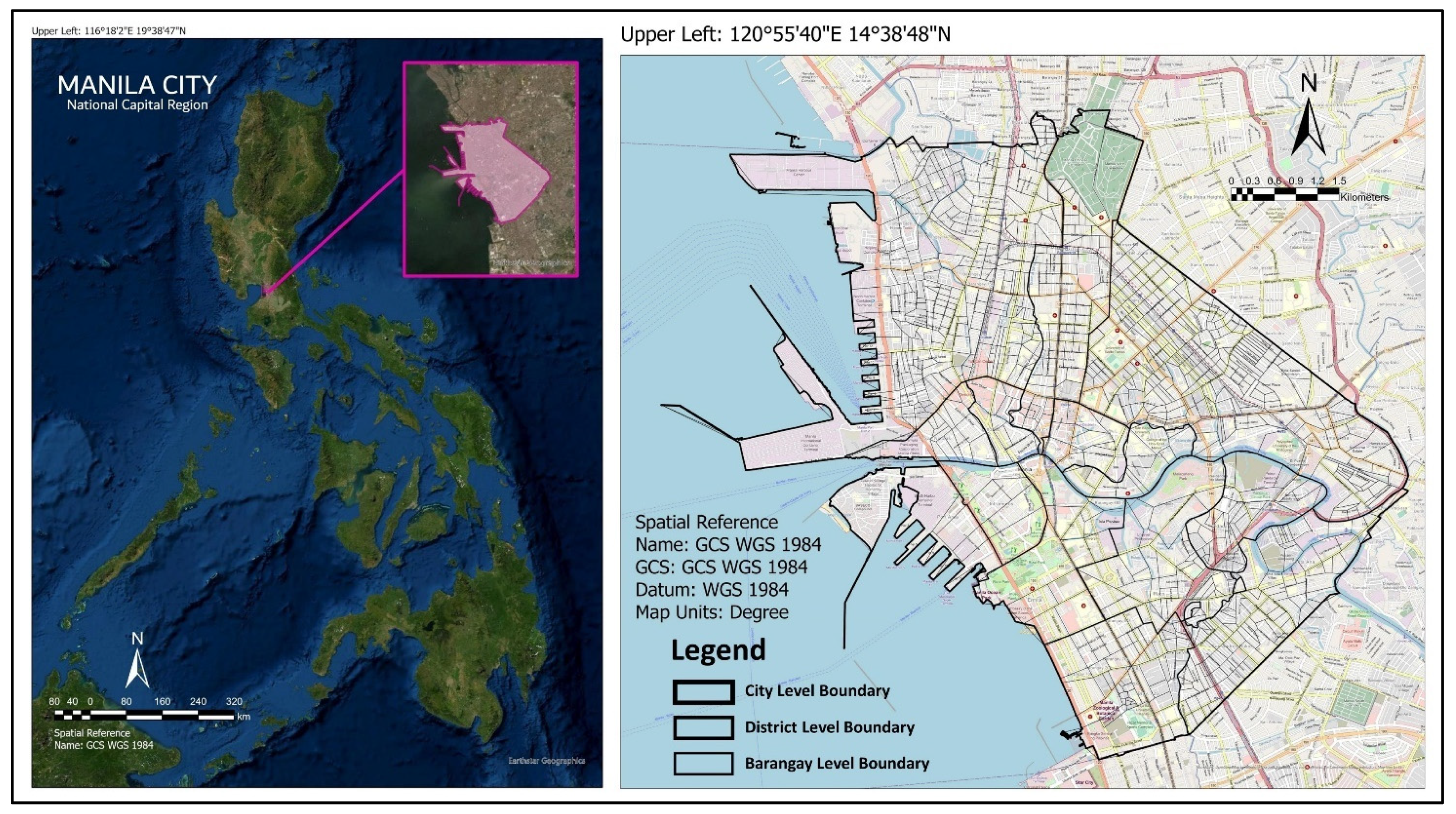The image consists of two side-by-side maps of Manila City and its National Capital Region. The left map, labeled "Manila City National Capital Region," is a satellite view presenting the blue ocean and green islands that compose the Philippines. An inset in the upper right corner of this map zooms in on the Manila City area. The map also includes a scale and a north-pointing arrow located in the bottom-right corner. 

The right map provides a detailed, zoomed-in view of Manila City, outlined with its streets and boundaries. It indicates specific coordinates: 120° 55' 40" E and 14° 38' 48" N. The legend, placed in the bottom-left corner, distinguishes city-level boundaries, district-level boundaries, and barangay-level boundaries through different line thicknesses. Additional information to the left of the city map includes references to the geographical coordinate system (GCS WGS 1984) and map units in degrees. The highlighted section of Manila City is marked in light purple/pink, further emphasizing its detailed street view.